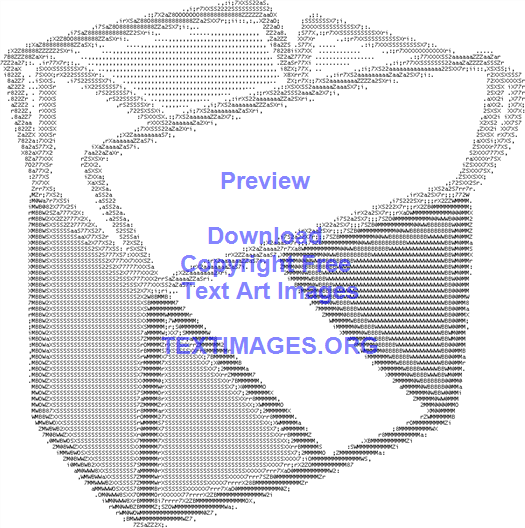This digital art image features an intricately designed open cardboard box created entirely out of small, black alphabets and numbers, meticulously organized to form a 3D rectangular shape with an open lid. The background of the image is white. Overlaid on this text-based artwork, centered in the image, is a purplish-blue semi-transparent text which reads: "Preview, Download, Copyright Free, Text Art Images, textimages.org." The box is depicted in a pixelated style, giving it a computer-generated appearance, yet the precision of using only text elements to create the visual is remarkable.